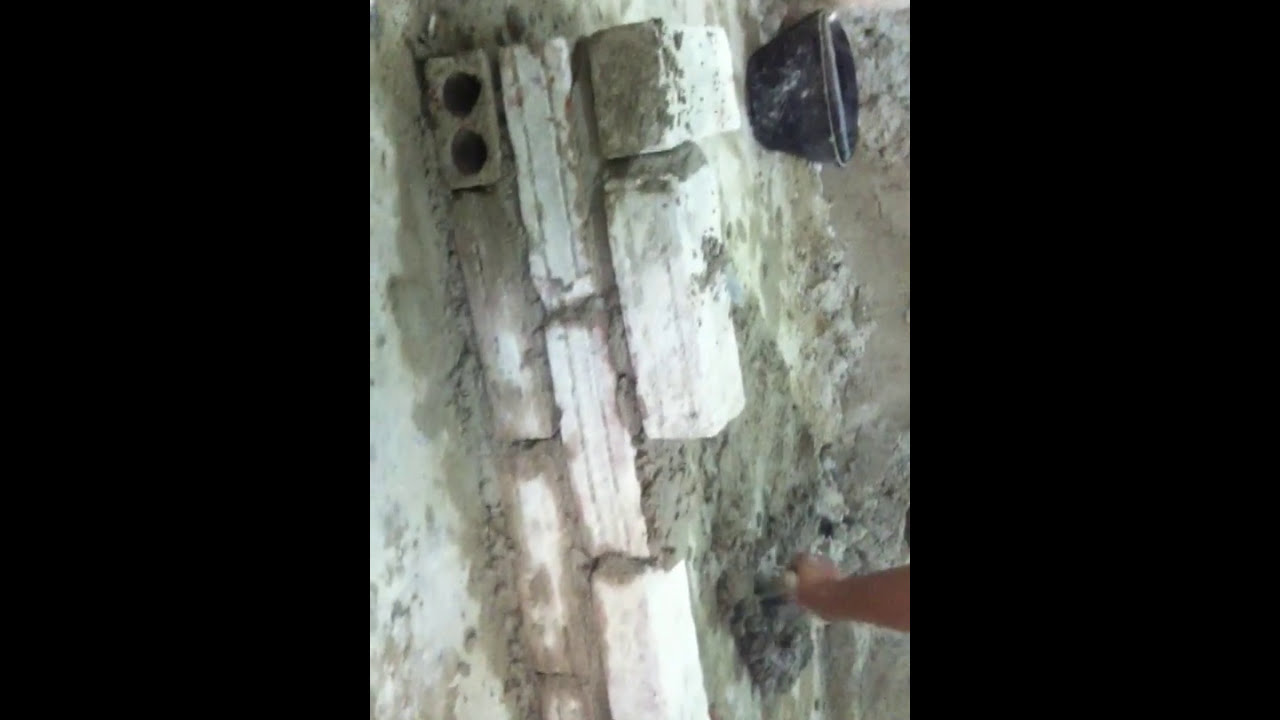The image captures the construction of a stone wall made of rectangular, white bricks, which, despite being rotated to the right, clearly displays a detailed masonry process. The thick gray mortar is spread between the bricks, with a significant portion being applied by a hand holding a trowel, which features a brown wooden handle and is located in the lower right corner of the image. The wall appears to be built from the ground up, with the scene presented in a vertical portrait orientation, further emphasized by black bars framing the image on both sides. A distinctive detail includes one brick in the top left corner that has two dark holes. Additionally, a black rubber or plastic bucket with a metal handle is situated in the upper right corner of the image, possibly used for carrying the mortar. The background reveals a floor that is predominantly flat and white, contrasting with a distant wall made of a caked brown material.